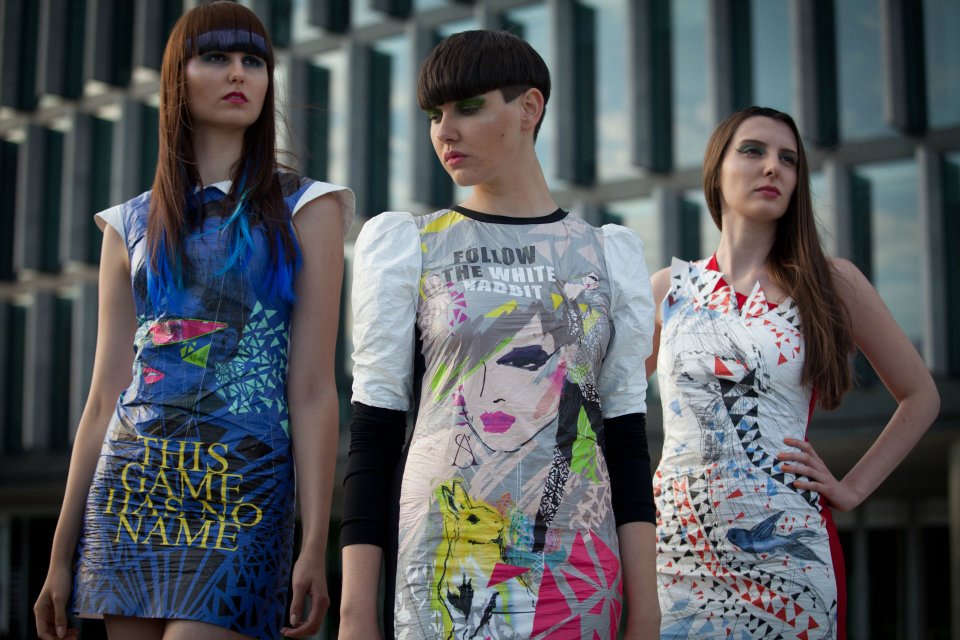In this vibrant color photograph, three female models stand confidently, each donning a unique mid-thigh dress that showcases distinct patterns and designs.

The first model on the left is dressed in a striking blue attire. Her dress features an intriguing blue text along the lower front that reads "This game has no name," complementing its blue and black textured skirt. White triangular patterns embellish the waist, while the top part flaunts white shoulders. Her straight brown hair is subtly accented with a matching blue streak across her front bangs, perfectly coordinated with her outfit.

In the center stands the second model, whose ensemble is a blend of white and gray. Her long-sleeved dress, adorned with puffed shoulders and a white trim around the neckline, displays an artistic illustration across the chest. The text "Follow the white rabbit" overlays the image of a woman with gray hair, complemented by a small painted rabbit in white and yellow near the abdomen. Accents of green and magenta add a vibrant touch to the dress. With her short dark hair and heavy makeup, she gazes slightly downward to her right, adding a touch of mystery.

The third model, on the right, wears a predominantly white dress with intricate reddish patterns and accents. The design includes a small gray fish and ribbon-like motifs, decorated with blacks and reds. The ruffled chest area and triangular ruffles around the front collar are subtly highlighted with red. Her long brown hair cascades down her back, completing her elegant look.

In the background, a vertical gray business building with side-by-side windows and slats adds an urban touch to the scene, contrasting with the chic, fashion-forward ensembles of the models.